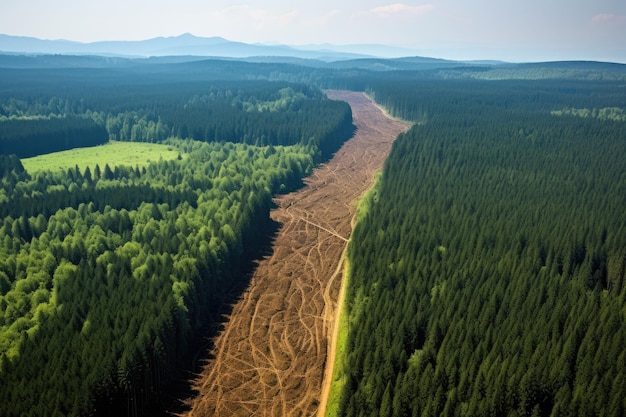This is a drone photograph captured in landscape orientation, providing a bird's-eye view of a large forested area. The image showcases two distinct sections of forest, separated by a wide, brown strip of land that appears recently cleared. On the right side of the photograph, a dense, dark green pine forest dominates the scene, while the left side features a forest of lighter green, deciduous trees, giving a softer, almost furry appearance due to their foliage. The cleared channel running from the bottom middle to the background is marked with visible trails and tire marks, suggesting recent development or forestry activity. In the distant background, the landscape transitions to a range of mountains, adding a dramatic backdrop to the scene. The contrast between the untouched forests and the sculpted, open strip creates a striking visual of both natural beauty and human impact.